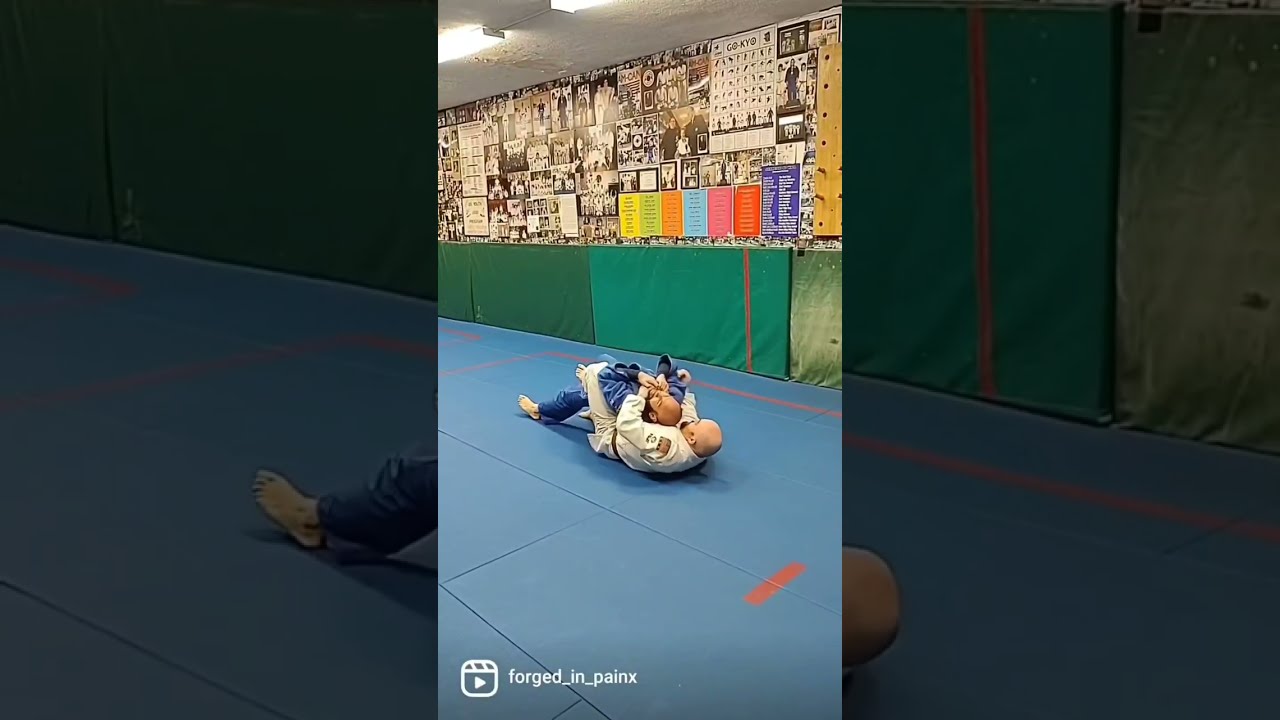The image features two men wrestling in a room designed for martial arts, with the action captured in a prominent vertical cell phone picture at the center. This central image is overlaid onto a faded, zoomed-in, and dimmer version of the same picture, creating a wide, horizontally-oriented aspect ratio. The men are dressed in karate gis—one in white, the other in blue. The man in white is on his back on a blue padded floor, wrapping his legs and arms around the man in blue, attempting to choke him from below. The room's furnishings include a padded section on the walls that runs waist-high and a mix of graphics and posters above. A dark green counter stretches along the wall, covering its base with what appears to be tarp-like material. Partial views of fluorescent lights hang from the ceiling, casting light over the scene. Additional visual elements include black and white pictures scattered across the upper wall amid the room's martial arts-themed decor.